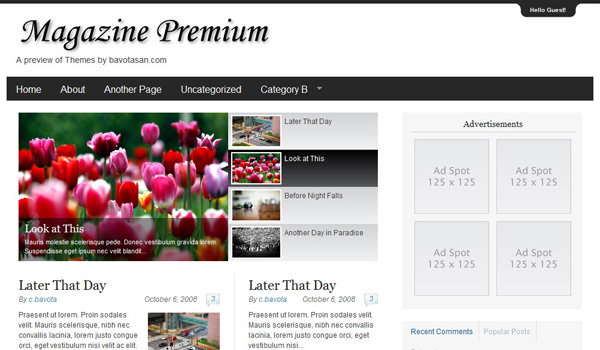This image is a detailed screenshot of a website template designed for a magazine, potentially focusing on floral themes. At the top, in a fancy font, it says "Magazine Premium" with a smaller subtext, "a preview of themes by bavotason.com." Below this header are clickable tabs labeled "Home," "About," "Another Page," "Uncategorized," and "Category B."

Central to this screenshot is a high-definition close-up of vibrant pink and red tulips, set against a blurred green background. To the right of this image is a sidebar with three smaller preview images titled "Later That Day," "Before Night Falls," and "Another Day in Paradise," offering snippets of visual articles.

On the left panel, similar previews appear, with the "Later That Day" title repeated, accompanied by brief text blurbs. The right side of the webpage features a dedicated advertisement section, marked by four blank squares labeled "Ad Spot 125 by 125," indicating potential ad placements. The template appears to be a flexible tool for creating or showcasing a floral-themed magazine website.